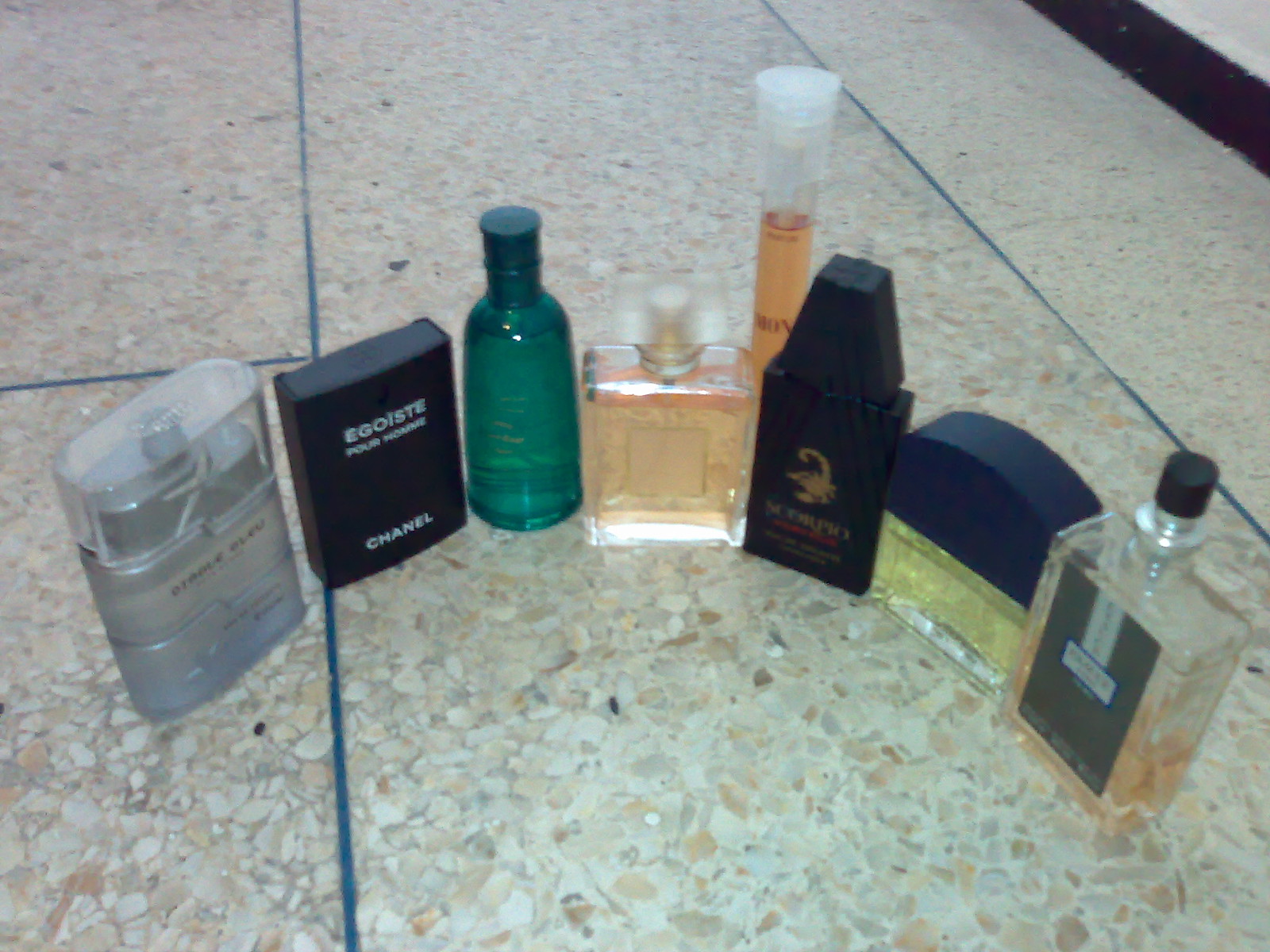This overhead photograph captures eight distinctive perfume and cologne bottles arranged in a semicircle on a detailed, textured tile floor composed of small, sanded rocks with black grout. The image is slightly blurry and out of focus, but the diverse characteristics of the bottles are discernible. Starting from the left, the collection begins with a silver, square-shaped bottle, possibly resembling a deodorant bottle with a clear lid and visible pump. Next is a black bottle labeled "Egoiste, Chanel." To its right, a green bottle with a plastic top and a transparent green liquid stands out. Following this, there is a clear bottle containing a peach-colored liquid and next to it, a tall, thin bottle that almost resembles a giant test tube with similar colored fluid. Further along, a black bottle decorated with a gold scorpion is visible. After that, a clear bottle with yellow fluid topped with a navy blue lid. Concluding the row is another clear bottle partially filled with peachy-orange liquid, missing its lid. The variety of shapes, sizes, and colors creates an intriguing visual display of scents.